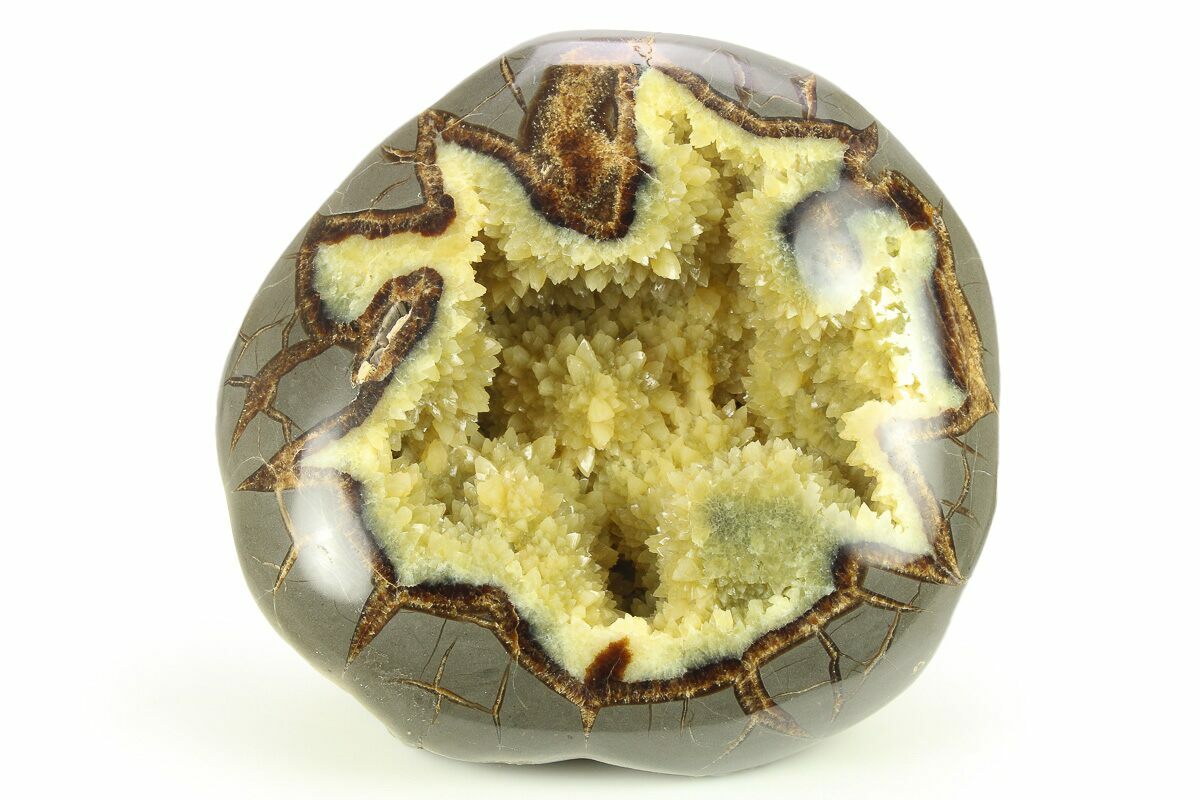This indoor photograph captures a highly polished geode resting on a flat, white background, intended as a showpiece or possibly a paperweight. The exterior of the geode is smooth and gray, adorned with brownish-gold veins and some milky white areas. The geode has been cut in half to reveal a cavity filled with glittering, pale yellow crystalline structures, resembling calcite or calcium deposits. These small, jagged crystals stand out against the gray mixed in at the base. The entire geode is approximately three to four inches high, presenting a stunning contrast between the polished outer surface and the raw, intricate crystalline formations within. The rock casts a slight shadow underneath, giving it a grounded appearance on the display surface.